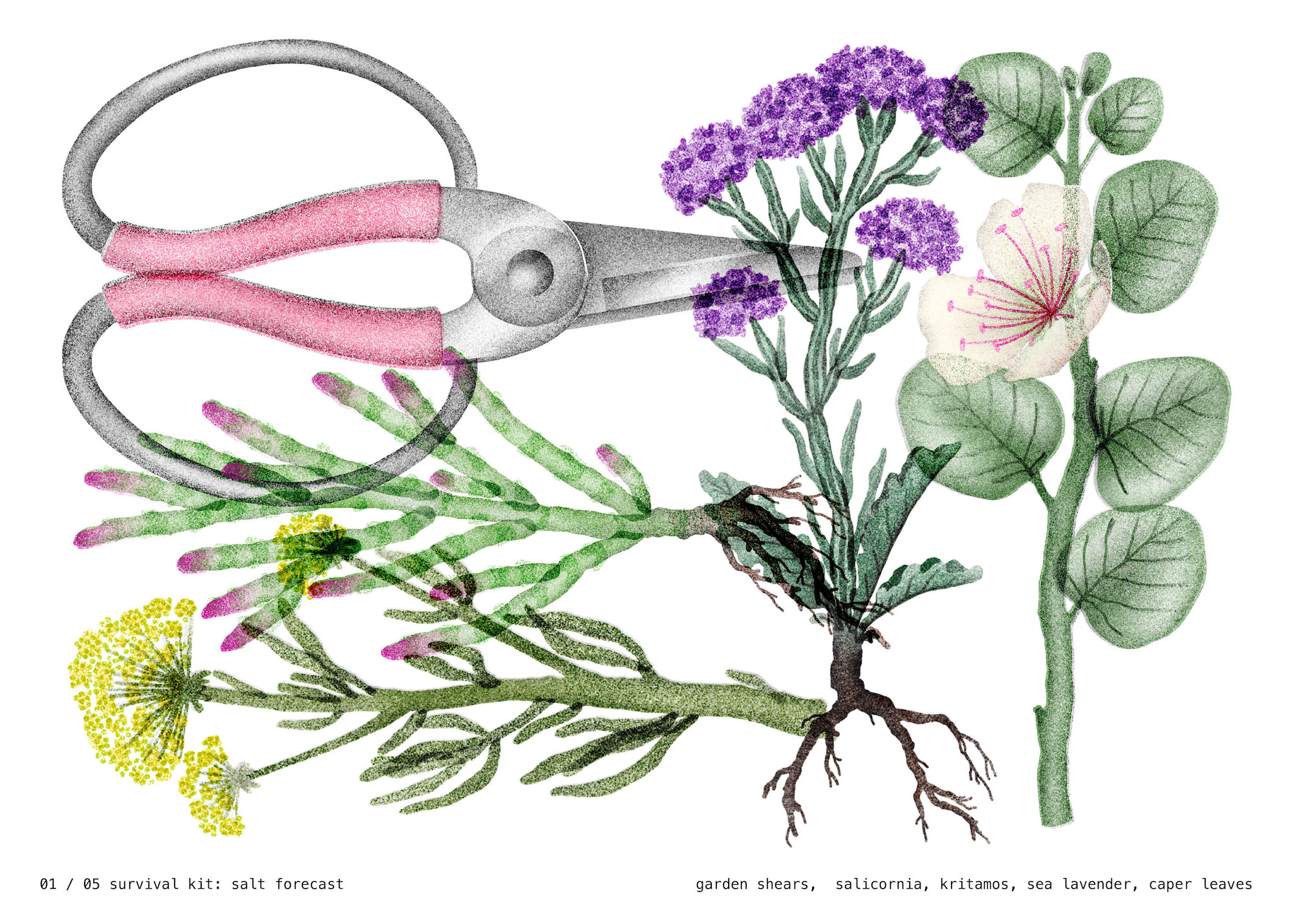This image, resembling a watercolor illustration, portrays a variety of plants alongside a pair of garden shears, suggestive of a botanical textbook illustration. The garden shears, positioned in the upper left corner, feature pink accents wrapped around their circular handles. These handles extend towards the left, with the blades reaching just beyond the center of the upper frame. Arranged in a vertical sequence beneath the shears are two plants, one with dark pink blooms and the other with yellow flowers. To the right, two upright plants are depicted. The plant on the left displays a portion of its root system along with purple pom-pom-like flowers atop its stem. Adjacent to it, the plant on the right has wide, almost round, silver-gray leaves and a white flower with pink stamens. Labels at the base of the illustration identify the species: Sea Lavender (blue flowers), Caper Leaves (silver gray), along with Salicornia and Critimus. The base of the image also bears the text "01-05 Survival Kit Salt Forecast."